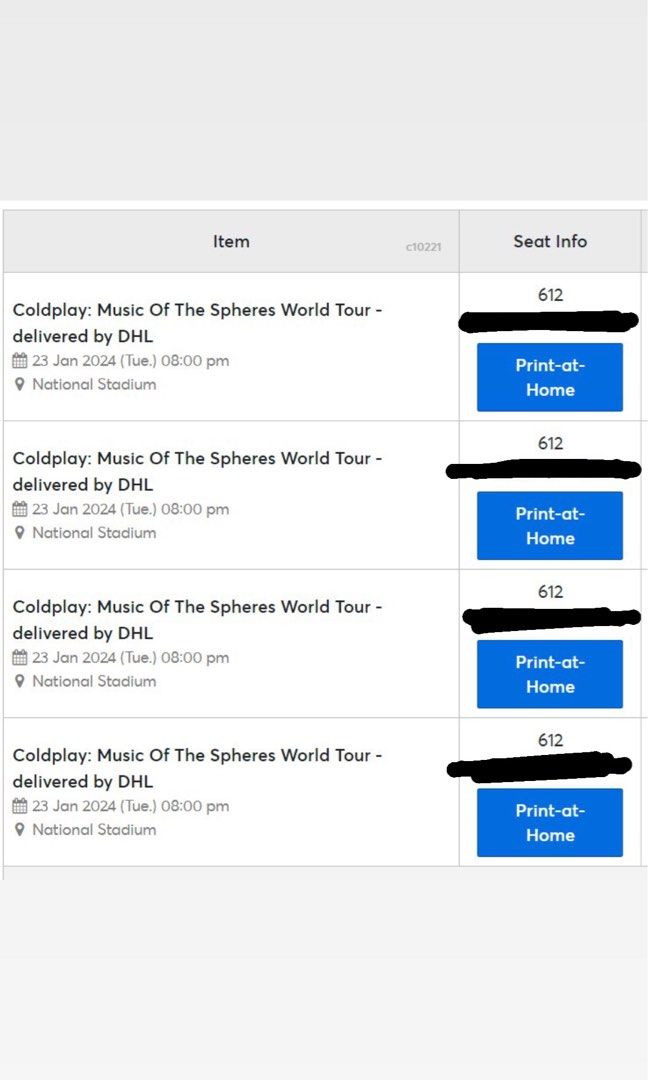In the image, we are looking at what appears to be a screenshot displaying ticket information for a concert. The layout is divided into two main columns: one labeled "Item" and the other "Seat Info." 

In the "Item" column, there are four entries, each detailing the event specifics:
1. "Coldplay, Music of the Spheres World Tour"
2. "Delivered by DHL, January 24th, 8 PM"
3. "National Stadium"
4. "Print at Home"

The information is repeated in all four entries, indicating that the screenshot shows four separate tickets for the same show.

These "Print at Home" tickets are marked within a blue box that has white writing on it, making it clear and prominent for the user. 

At the top of the image, there is a light grey box, which likely contains header information or navigation options, although these details are not specified. The overall background of the screenshot is white, with the text displayed in black for readability.